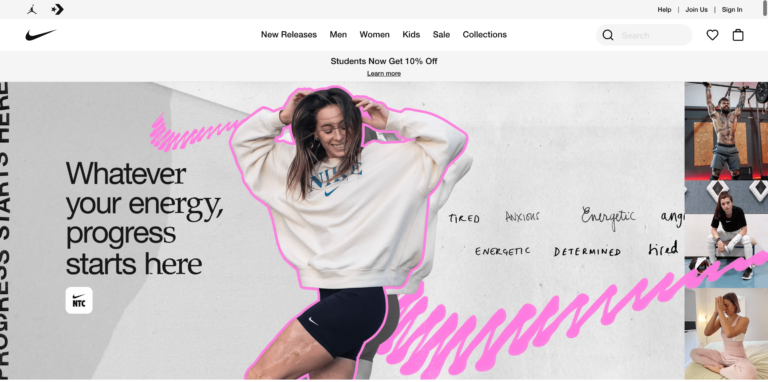Screenshot of the WeaveNike.com homepage showcasing various interface elements and a promotional banner. 

At the top, a grey navigation bar spans the width of the page. On the left side of this bar, the black Michael Jordan Jumpman logo is displayed, alongside a thick arrow pointing to a small star. On the right side, there are links labeled "Help," "Join Us," and "Sign In."

Below this bar, another section features a white background. To the left, the black Nike swoosh logo is prominently displayed. Centralized in this section are menu options reading "New Releases," "Men," "Women," "Kids," "Sale," and "Collections." Next to these, there is a search icon represented by a magnifying glass, a heart icon for favoriting items, and a shopping bag icon for the cart.

The main banner has a pinkish-grey background and showcases a white woman positioned slightly left of center. She is wearing a white Nike sweatshirt with a blue Nike swoosh logo on it and black tight shorts with a Nike swoosh emblem. The woman has light brown hair, has her hands raised cheerfully, and is smiling energetically.

On the left side of the banner in black text, it says, "Whatever your energy, progress starts here." Below this, words like "Tired," "Anxious," "Energetic," and "Determined" are written, highlighting different states of mind or energy levels. Additionally, the banner features still images of people working out in Nike apparel, reinforcing the message that Nike gear is essential for workouts.